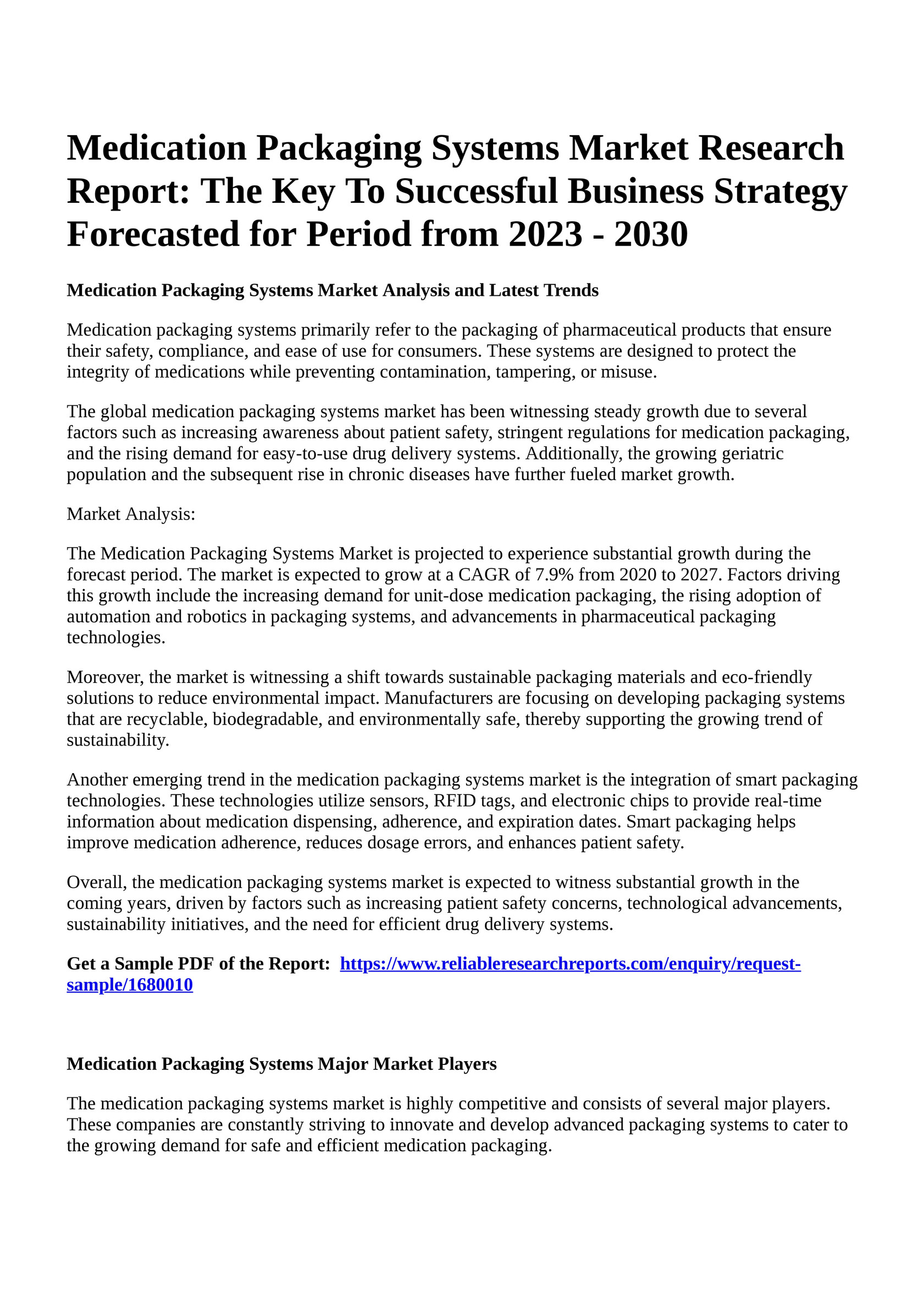The image displays a page from what appears to be an article titled "Medication Packaging Systems Market Research Report: The Key to Successful Business Strategy Forecasted for a Period from 2023 to 2030." The section title reads "Medication Packaging Systems Market Analysis and Latest Trends." The page contains several short paragraphs of text that are difficult to read due to their small font size. At the bottom of the page, there is a clickable link prompting readers to "Get a sample PDF of the report," and an additional section titled "Medication Packaging Systems Major Market Players," which includes a paragraph elaborating on this subject.